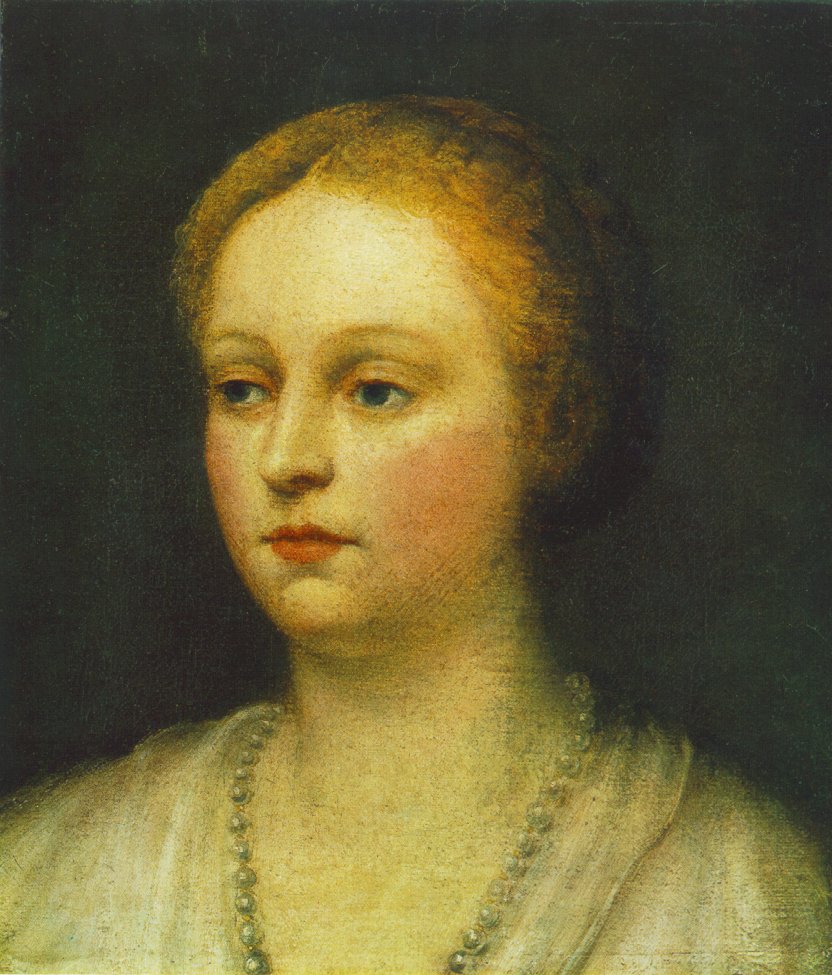The image is a detailed oil painting portrait of a woman, likely from the Renaissance period, depicted from the upper chest upwards. She is facing and looking slightly to the left with slightly lidded, serious eyes that give her an almost stern, tired appearance. Her rounded face is accentuated with a subtle pink blush on her cheeks and light red lipstick. She has thin, blonde eyebrows and full but small lips. Her hair, which seems to be a nuanced reddish-blonde, is pinned up neatly behind her head.

The woman is adorned with a pearl necklace, visible on either side of her neck where the painting allows. She wears a white garment that some perceive as having a teal tint, indicative of traditional attire from the 1500s to 1600s period, potentially suggesting British origins. Her neckline is deep, and her neck appears thick.

The background is a textured mix of dark colors, predominantly black and gray or dark brown, showcasing visible brush strokes that add to the painting's classical and somewhat unfinished, yet charmingly raw aesthetic. This enhances the old-world charm of the portrayal, emphasizing the striking contrast between the finely detailed subject and the rudimentary backdrop.